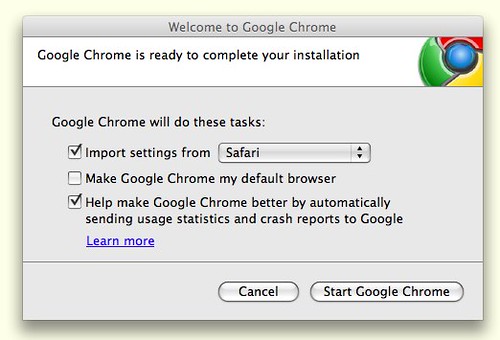The image features a dialogue box with a gray header that reads "Welcome to Google Chrome." The word "Welcome" starts with a capital W, while "Google" has a capital G and "Chrome" has a capital C. Below the header, a white rectangular box contains the message: "Google Chrome is ready to complete your installation," accompanied by the Google Chrome logo. The logo consists of a blue circle at the center, surrounded by a broken ring of green, red, and yellow segments, representing Google's signature colors.

Underneath the installation message, there's a section outlining several options for the user. The first option is to "Import settings from," with Safari as the pre-selected browser. This option is indicated by a box with a checkmark. The second option, "Make Google Chrome my default browser," is displayed with an empty checkbox, signifying that the user has not chosen this setting. The third option, "Help make Google Chrome better by automatically sending usage statistics and crash reports to Google," is marked with a check, and a "Learn More" link in blue text is provided for additional information.

A horizontal gray line separates these options from the action buttons at the bottom of the box. Two buttons are present: "Cancel" on the left and "Start Google Chrome" on the right.